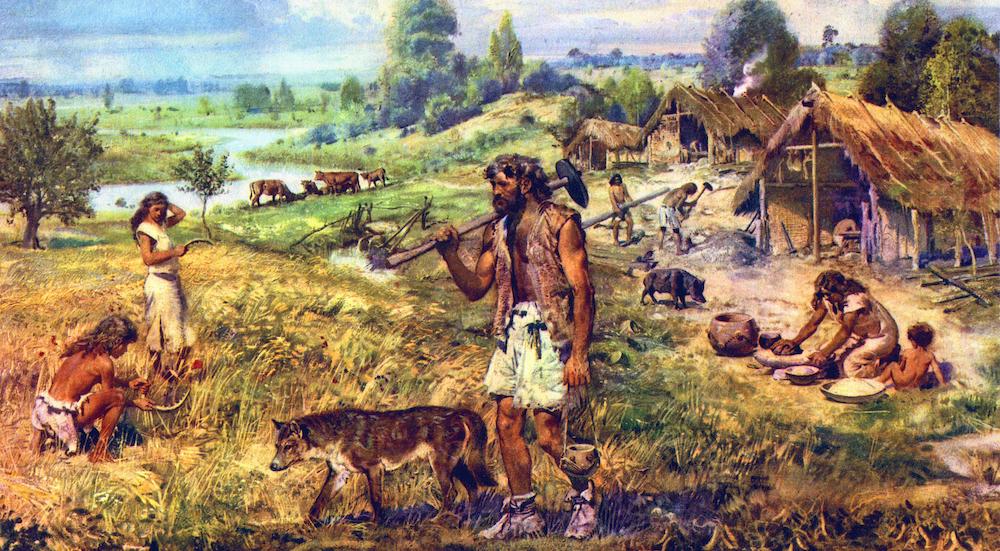The painting depicts a prehistoric community engaging in various activities around a cluster of thatched huts with simple support poles. Prominently in the foreground, a rugged, bearded man with shaggy hair stands wearing an open vest made of hide, shorts, and moccasins tied around his feet. Over his shoulder, he carries a long pole equipped with a metal tool, hinting at early metal use. Beside him, a wolf or early domesticated dog walks, indicating a period during the domestication of canines.

To the left, a person in a loincloth squats beside a girl wearing a skirt and a brown top, while two cows can be seen by a pond in the distance, contributing to the rural setting. On the right side, a cluster of thatched huts stretches from the middle to the right edge of the scene. Within one hut, a woman crouches, grinding something on a stone with a naked toddler beside her and a pig nearby. 

Scattered through the painting are other figures: a man chopping with an axe and another holding what appears to be a wooden board. The vivid details of people in ragged clothing, alongside clear distinctions of their various daily tasks, bring this ancient community to life, showcasing a moment in time from early human civilization. Trees and grassland create a serene backdrop, completing this rich depiction of prehistoric society.